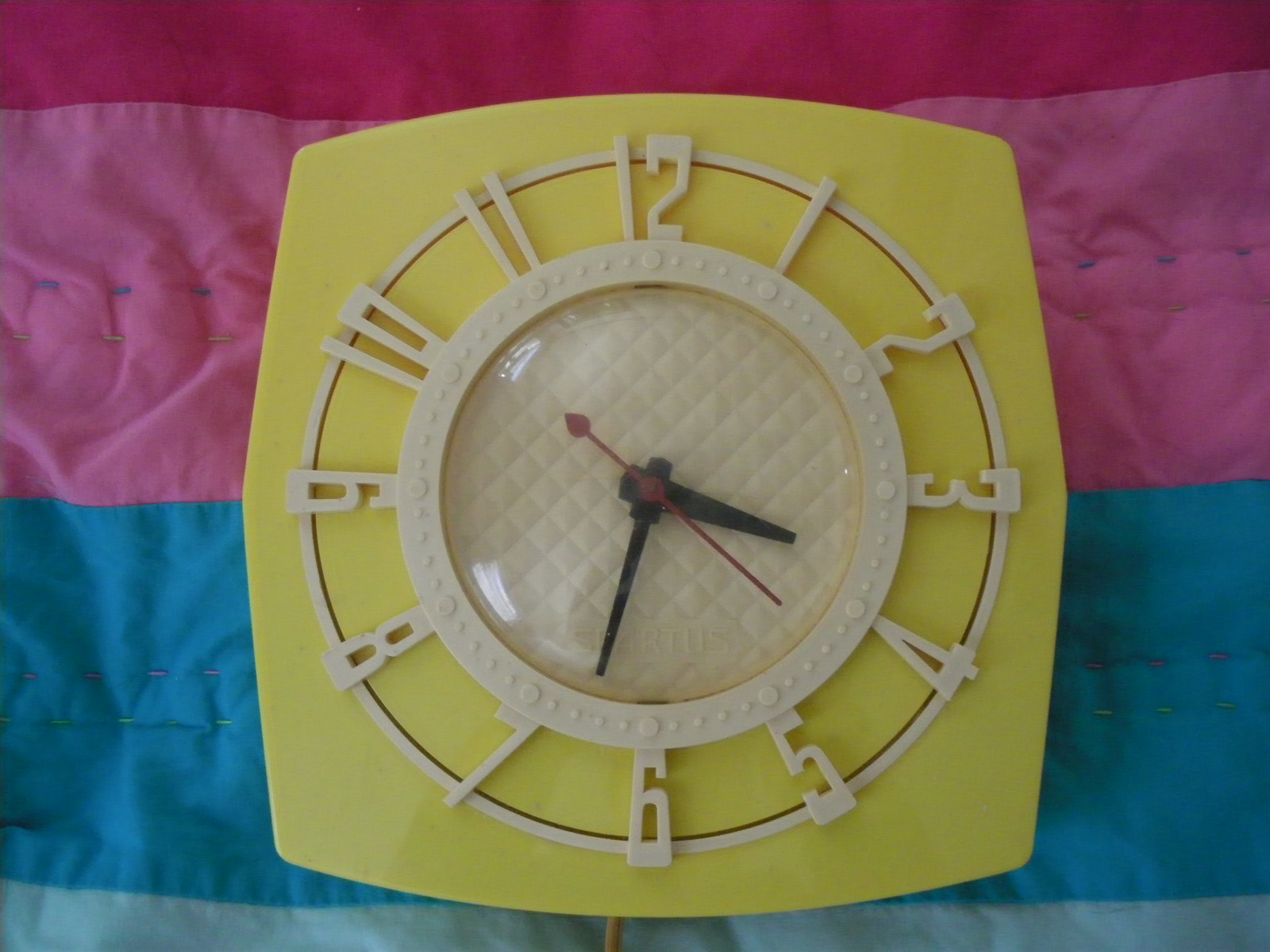A square, yellow clock features prominently in the image. The clock's design includes white, three-dimensional numbers around its perimeter, which are slightly protruding, giving them a more tangible appearance. At the center of the clock, there's a distinctive, multi-bowled, white, diamond-shaped plastic section with a bubble over it. This central section houses the clock hands: thick and short hour and minute hands, and a thin red second hand, which is currently positioned at the 22-second mark. The time displayed is 3:33. The background of the image shows the clock resting on a patterned blanket or quilt with horizontal stripes in various colors—magenta on top, followed by pink, dark blue, and baby blue at the bottom. Additionally, a small, dirty orange wire is visible, extending from the bottom of the clock.